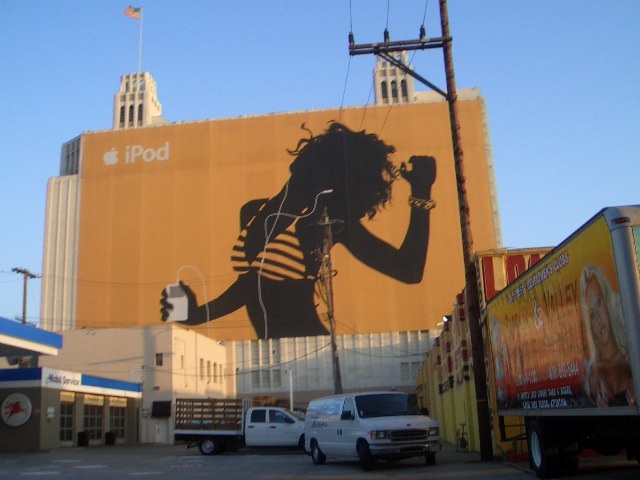This image captures a bustling city scene dominated by a large billboard attached to a stone building, with a clear blue sky above. The billboard features an orange-yellow background with the Apple icon and "iPod" in white text in the upper left-hand corner. The central figure on the billboard is a black silhouette of a woman in motion, her hair flowing as she tilts her head back. She is wearing a striped bikini in shades of orange and black that complement the billboard's background, and an orange bracelet on her left wrist. In her right hand, she holds a white iPod with a gray screen, and the white earphone wires are visible, trailing from her ears to the device. Below the billboard, the cityscape includes several white vehicles, notably a van and a commercial truck with a trailer, along with a nearby commercial building featuring yellow paint and red lettering. An American flag can be seen atop the building, emphasizing the urban American setting. Additional details include a building with a "Mobile Service" sign on the lower right, displaying white and blue stripes on its roof and a series of glass-paneled garage doors.